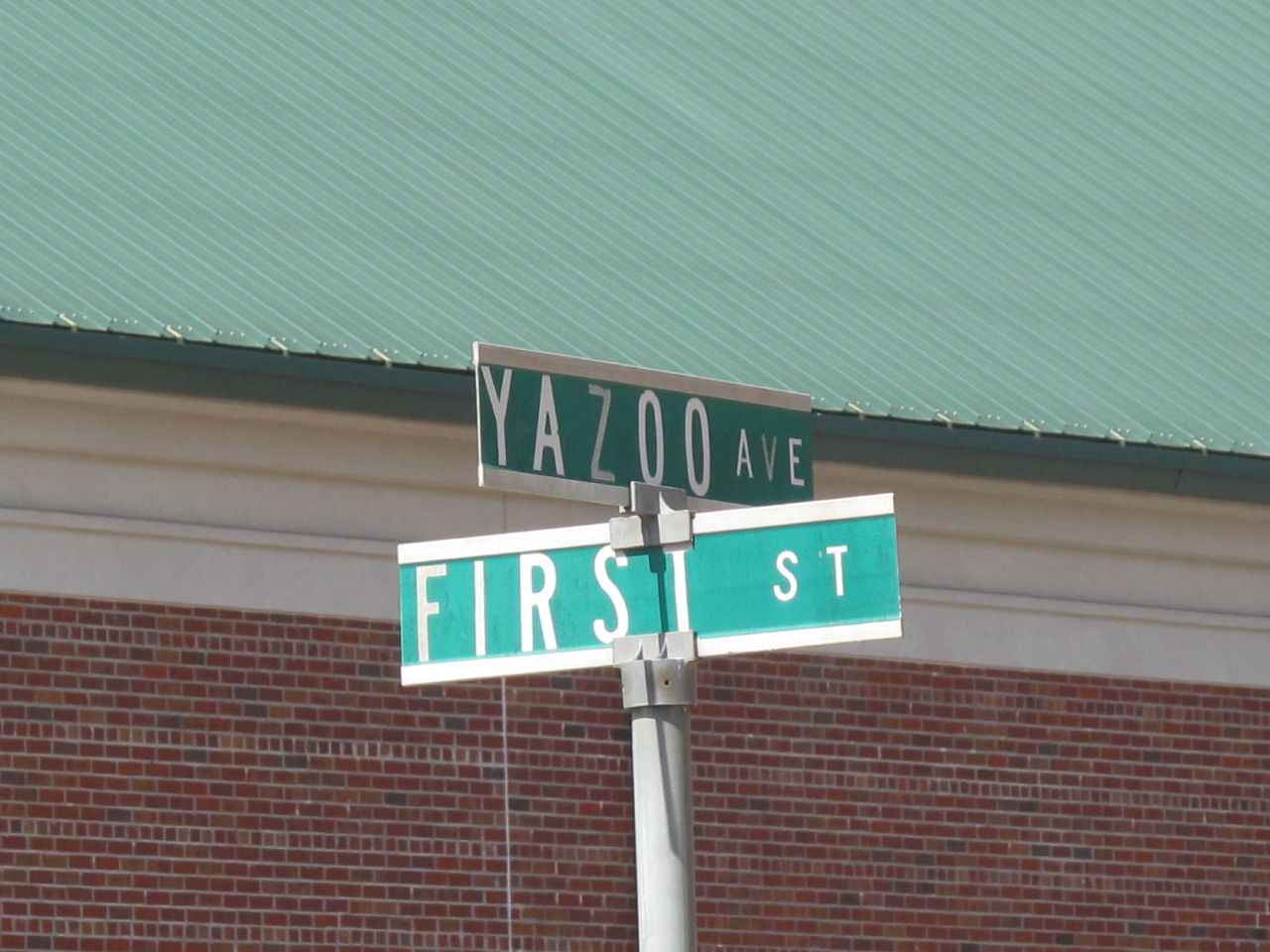A detailed description of the image features a red brick building with a light green metal roof. Between the roof and the brick structure, a beige trim of metal or steel adds a distinctive accent. In front of this building, a silver post holds two street signs. The sign facing forward reads "FIRST STREET," while the sign positioned behind it is labeled "YAZOO AVENUE." This image captures a crisp and well-defined urban scene, highlighting both the architectural elements and the intersection of two streets.